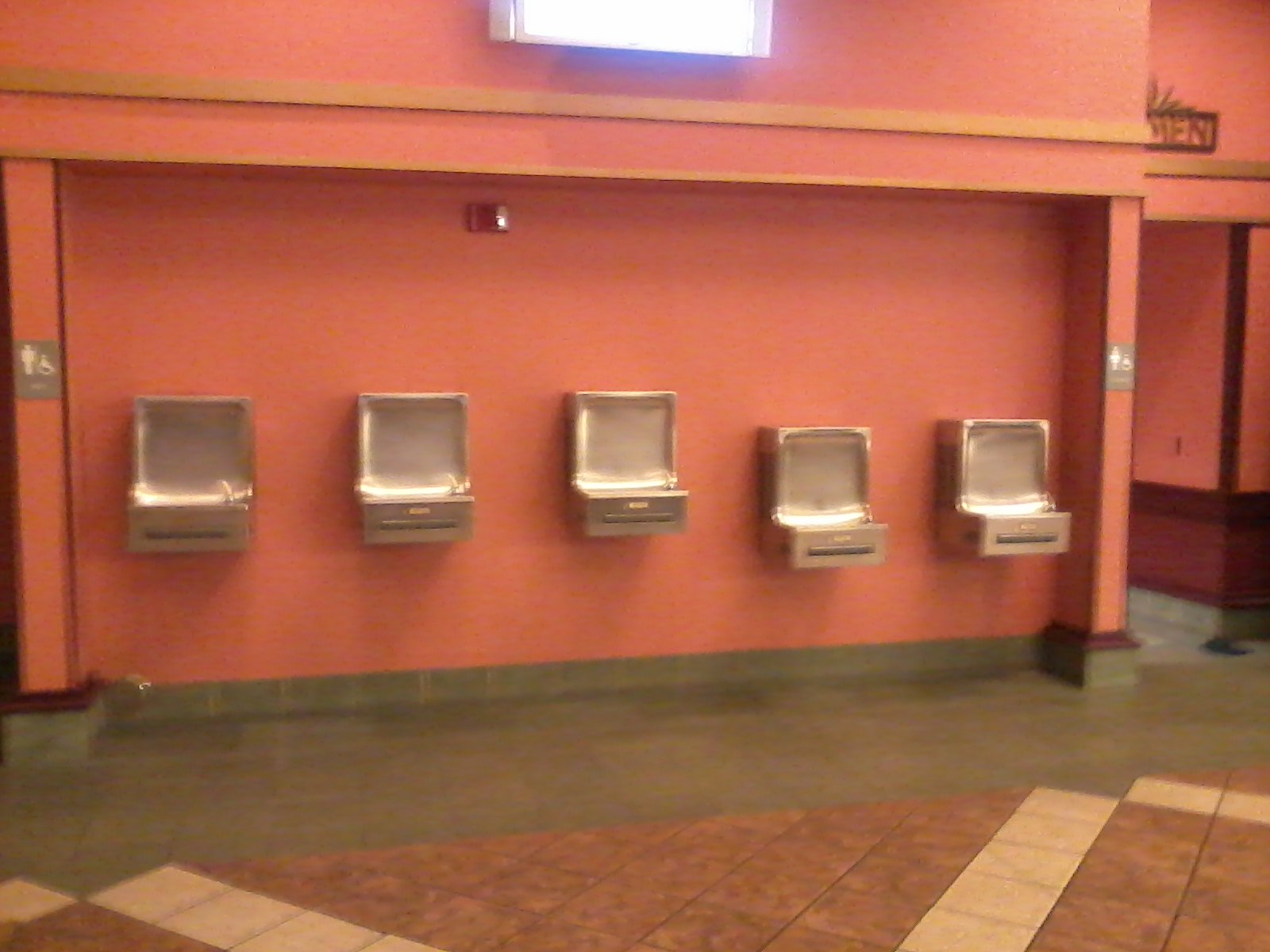In the brightly lit interior, five drinking fountains are aligned horizontally against a dark peachy, salmon-pink wall with gold trim. The fountains, which have a shiny steel rectangular design with a pooling lip and a long gray push bar, are arranged with three placed higher on the left, nearer to the men's bathroom, and two slightly lower on the right, closer to the women's bathroom. Above the fountains, a central white light illuminates the scene. The floor beneath the fountains consists of gray tiles, transitioning into a patterned area of terracotta and tan tiles with beige and light brown accents. On the left, a column displaying the men's room sign flanks the fountains, while on the right, a column shows part of a women's room sign, leading to the corresponding restroom doors. The entire setup, both functional and unexpectedly amusing, captures a blend of humor and functionality in its unusual arrangement.